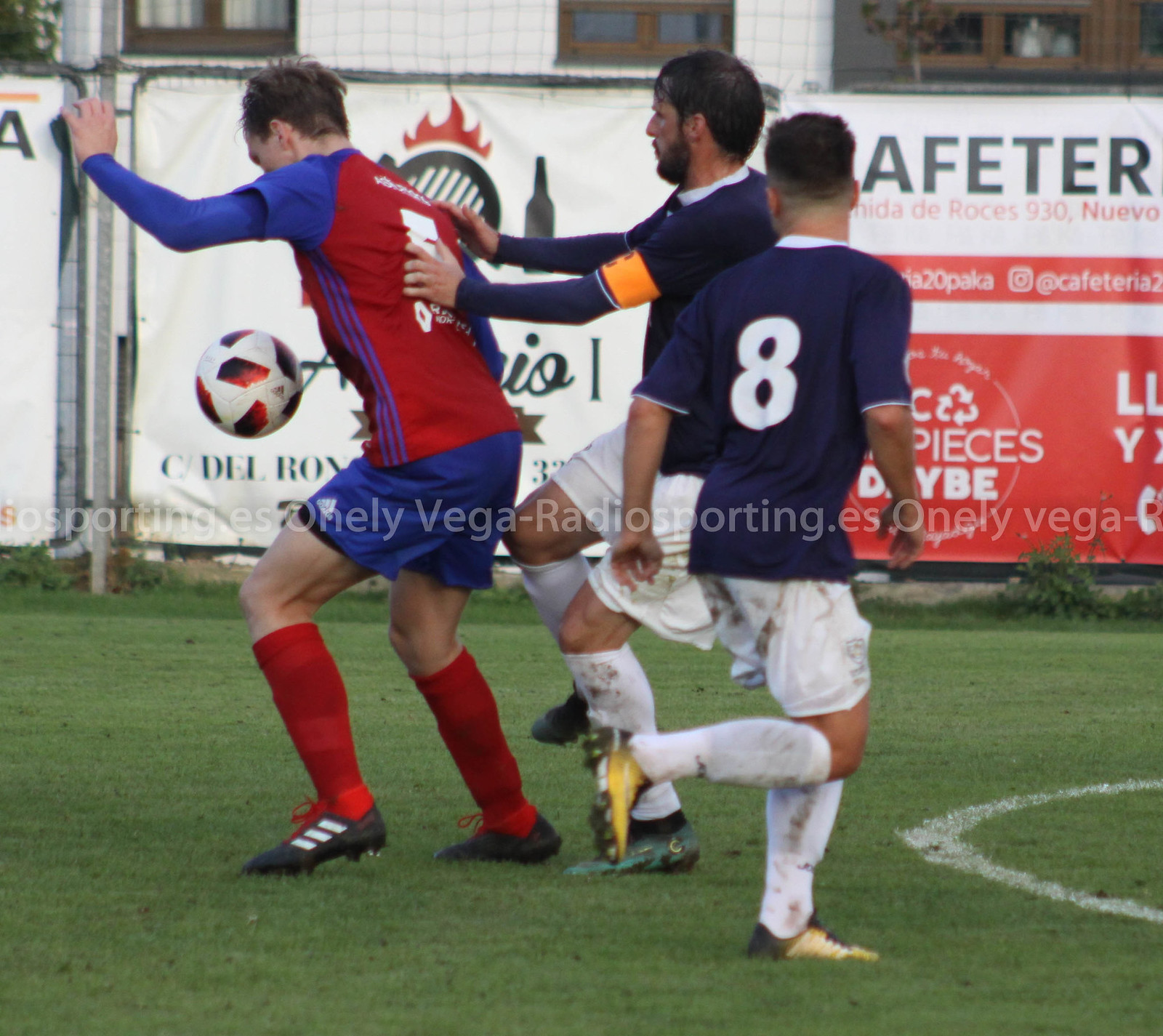In this dynamic outdoor photograph, three male soccer players are intensely engaged in a match on a vibrant green field, each donning distinctive jerseys; two in blue and white, and one in red and blue. The focal point is the player on the right, sporting a number eight jersey, white shorts, long socks, and cleats, with one foot airborne, indicating a powerful motion. The central player, mid-stride, stretches out his hands as if to steady himself against the player on the left, who is poised to kick a soccer ball that hovers near his abdomen. This player, with his left hand and arm extended and left leg forward, appears ready to strike the ball with his knee. The field is marked by white paint, adding to the competitive atmosphere. In the background, tall wall placards with various advertisements, one partially reading "Something Aster" and another "Pieces Baby" in red, add to the scene's commercial backdrop while an additional symbol or icon completes the setting. The captured moment highlights the active engagement and spirited interaction among the players.